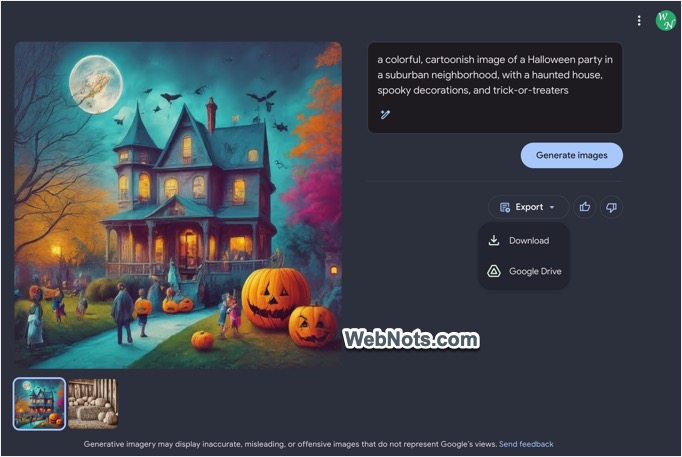A vibrant, cartoonish Halloween scene unfolds in this AI-generated illustration. Central to the image is a spooky haunted house, with eerie decorations that immediately catch the eye. Above, a full moon casts a ghostly glow, silhouetting a flock of crows in flight. On the ground, cheerful trick-or-treaters move from house to house, their costumes bringing life to the dark ambiance. The yard features several creepy, carved pumpkins with menacing faces, adding to the frightful atmosphere.

Surrounding the haunted house are three distinct trees: one withered and bare, another completely devoid of leaves, and a third unexpectedly blooming, providing contrast and depth to the scene. The color palette is a striking blend of blue, orange, yellow, grey, black, and green, enhancing the image's festive Halloween spirit.

In the lower corner, user interface elements like a like button, a dislike button, and export and download options hint at the digital and shareable nature of the creation. The entire composition suggests a lively Halloween party set in a suburban neighborhood, captured perfectly in animated form.